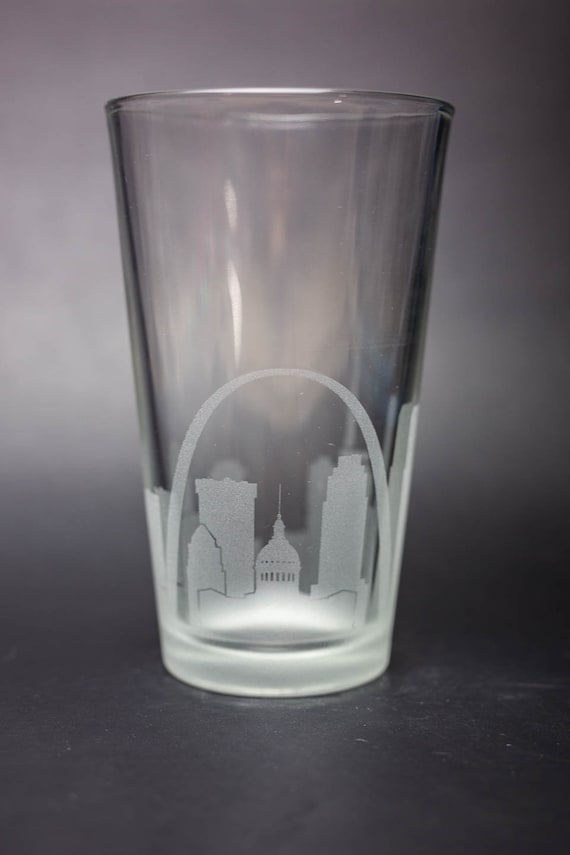The image depicts a clear, empty drinking glass positioned against a gray, vertically oriented background. The glass itself is simple and round with a flat bottom. On the exterior of the glass, there is an etched cityscape design featuring four buildings, one of which appears to resemble the Capitol building with its distinctive dome and pointed top. The other buildings vary in height and shape. An arched element is also part of the design. The background of the photo transitions from a darker gray at the bottom, suggesting a tabletop, to a lighter gray towards the top. The glass is somewhat reflective, indicating the presence of a nearby light source.